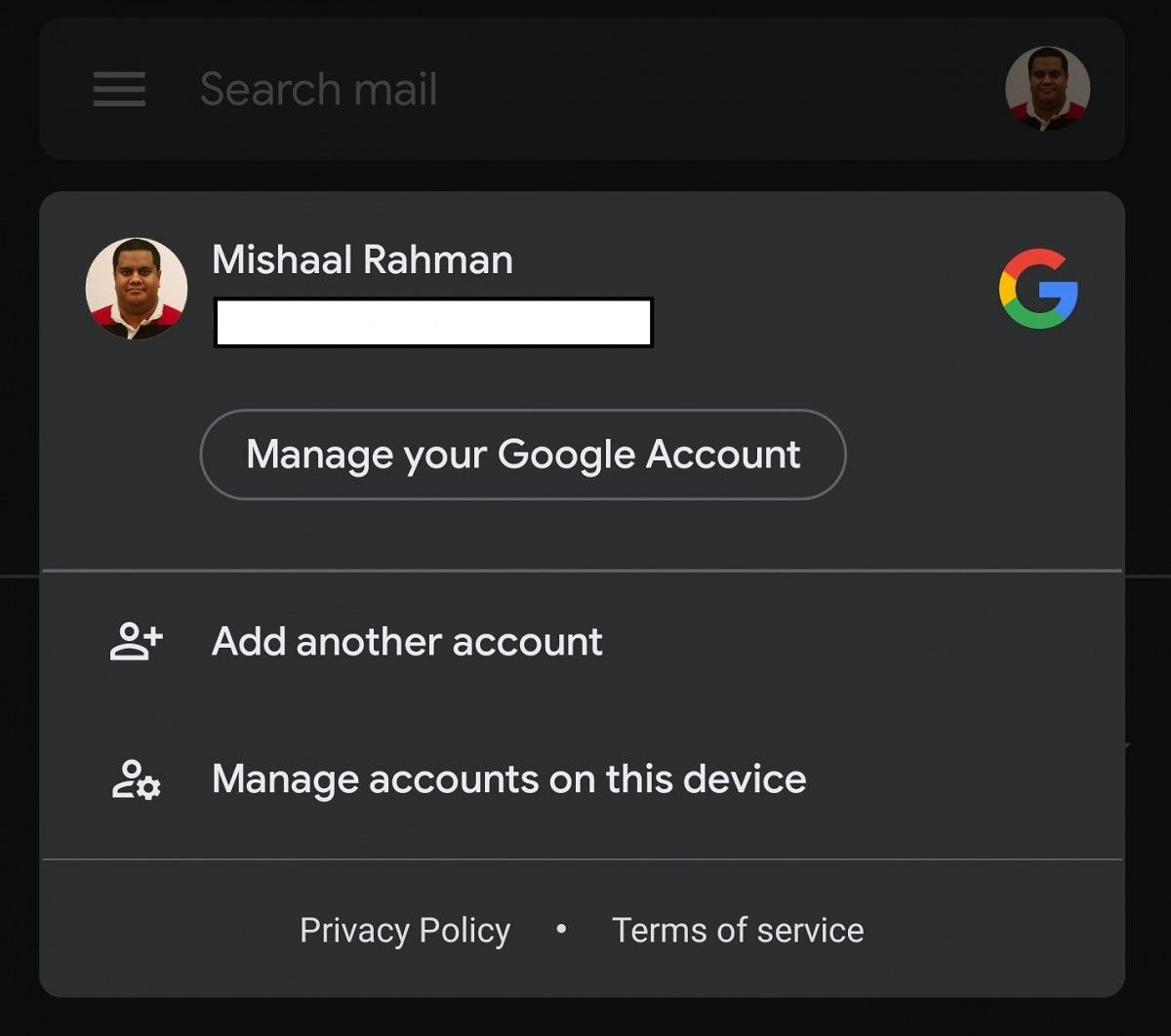This image showcases the management interface of a Google account with a completely black background. In the upper left corner, three medium gray horizontal lines indicate the menu button. Adjacent to it, "Search mail" is displayed. In the upper right corner, there is a profile picture of the account holder, presumably Michelle Rahman. Below the "Search mail" bar, the same profile picture is repeated with the name "Mishaal Rahman" (spelled M-I-S-H-A-A-L R-A-H-M-A-N) in white font. 

Directly below the name, a search bar is visible but remains empty. To the right of this search bar, the Google "G" logo is present. Underneath the name "Mishaal Rahman," the text "Manage your Google Account" appears, enclosed within a circle and also in white font. Further down, there is an icon indicating adding a person, accompanied by the text "Add another account."

The following section contains a person icon with a settings gear next to it, and the text "Manage accounts on this device" to the right. At the very bottom of the image, two links are provided, one leading to the "Privacy Policy" and the other to the "Terms of Service," both related to Google.